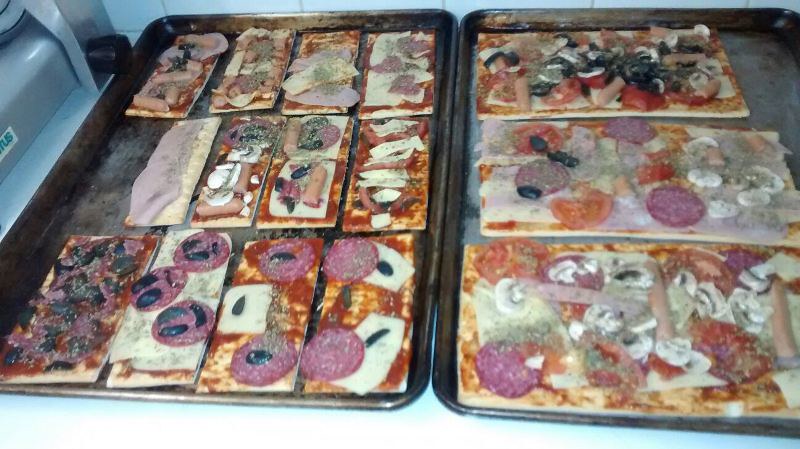The image showcases two silver baking pans placed side by side, each containing a variety of uncooked flatbread that resemble rectangular slices of pizza. The baking pan on the left features three large flatbread squares adorned with toppings like pepperoni, black olives, various meats, and cheese; these appear frozen and unbaked. The right baking pan holds twelve smaller pieces of flatbread arranged in three rows of four. Each slice features a mix of toppings including cheese, pepperoni, black olives, and meat, though one slice notably has minimal toppings. Additionally, some slices seem to have tomatoes and sausage, while one stands out with no toppings but a dash of meat. The overall setting includes a blue table and background with blue tile work visible.